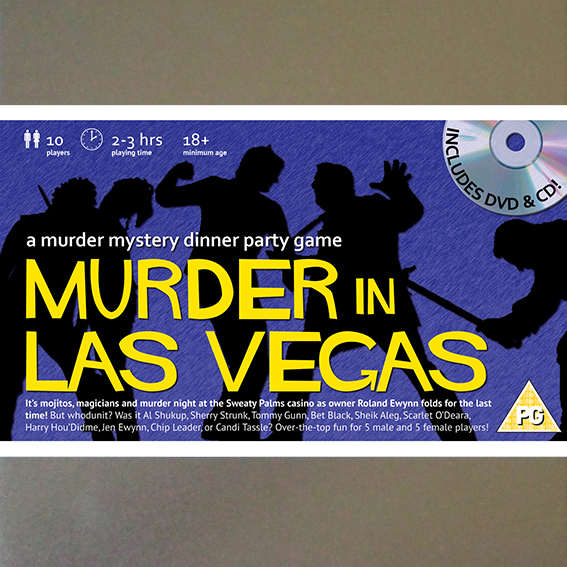This image appears to be an advertisement for a murder mystery dinner party game titled "Murder in Las Vegas." The background is primarily blue, featuring the silhouettes of six figures, five men and one possibly a woman, depicted entirely in black. Some figures are holding objects that appear to be weapons such as a hammer, knife, gun, and sword. Bold, bright yellow letters span across the center of the image, stating "Murder in Las Vegas." Above in white text, it reads "A murder mystery dinner party game." Below this, it provides the game's setting: "It's Mojito's Magicians and Murder Night at the Sweaty Palms Casino as owner Roland Ewan folds for the last time. But who done it? Was it Al Shookup, Sherry Stunk, Johnny Tiny Gun, Bet Black, Sheik Oleg, Scarlett Odeira, Harry Houdini, Jen Edwin, Ship Leader, or Cassie Tassel?" It is described as over-the-top fun designed for 5 male and 5 female players. Additional details include a yellow triangle in the lower right-hand corner indicating the game is rated PG, while the upper left-hand corner specifies it is meant for 10 players, with a playing time of 2-3 hours and a minimum age of 18. The upper right-hand corner features an image of a DVD and CD with black text noting "Includes DVD and CD." The advertisement's color scheme is varied, incorporating white, purple, black, yellow, gray, pink, and orange.